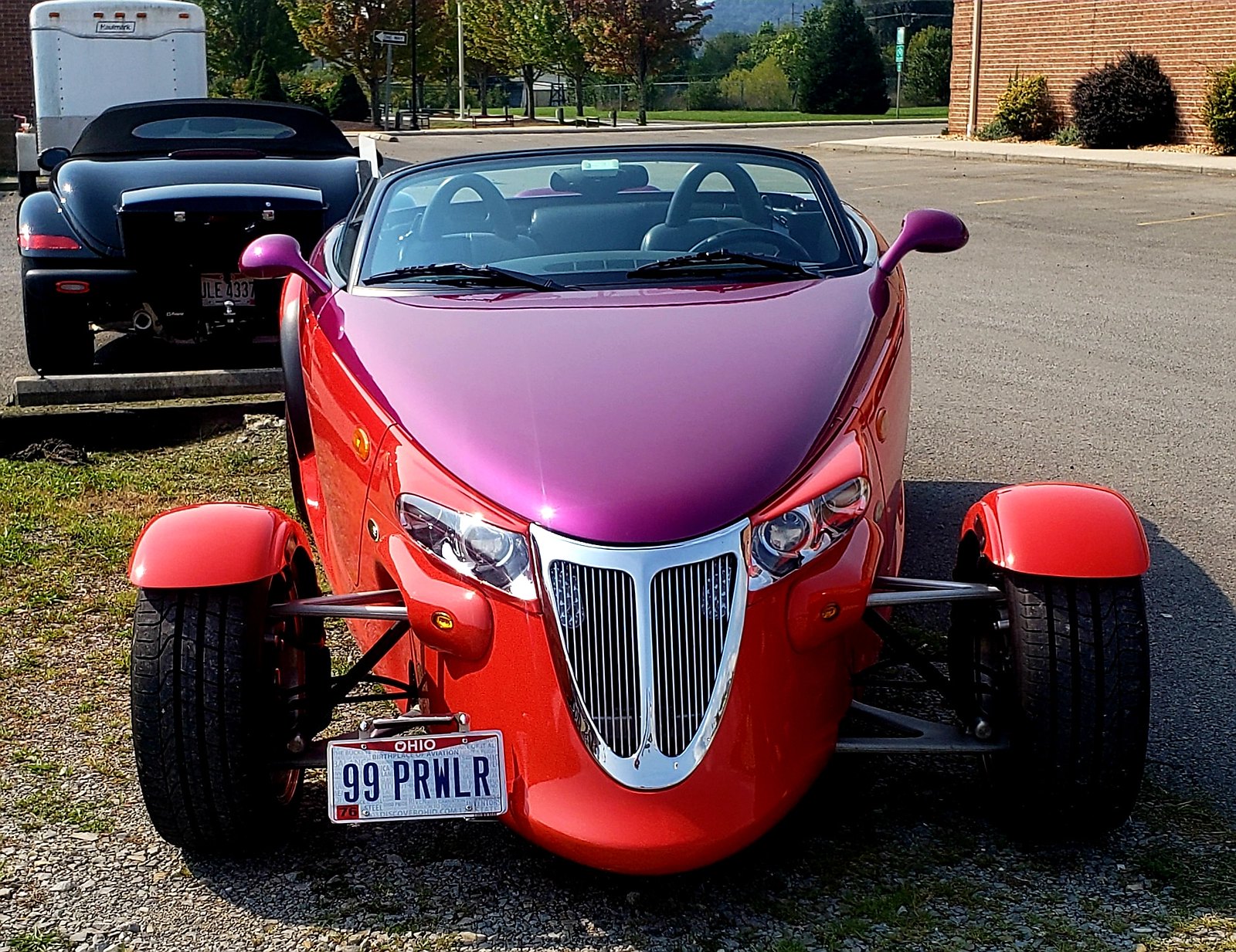The photograph features a striking 1999 Plymouth Prowler, a hot rod-styled car, prominently displayed from the front. The distinctive vehicle boasts a purple hood contrasted with a fire engine red body. Its front end is particularly eye-catching, with a chrome grille resembling a mouth, reminiscent of the Joker's smile, flanked by headlights. The front tires are mounted on exposed struts, each adorned with wide motorcycle-like fenders that give the impression of floating independently from the car's body.

A unique detail is the car’s red and white license plate located on the left side, reading "Ohio 99 PRWLR," a nod to the car's model year and the Prowler name. Enhancing its hot rod persona, the vehicle features a compact windshield with small side mirrors extending outwards.

In the background, the rear of another Plymouth Prowler is visible, as well as a white trailer. The setting is an open area near a parking lot, bordered by a red brick building, with trees, a street sign, and additional streets in the distance. The scene suggests a car show or gathering of automotive enthusiasts.